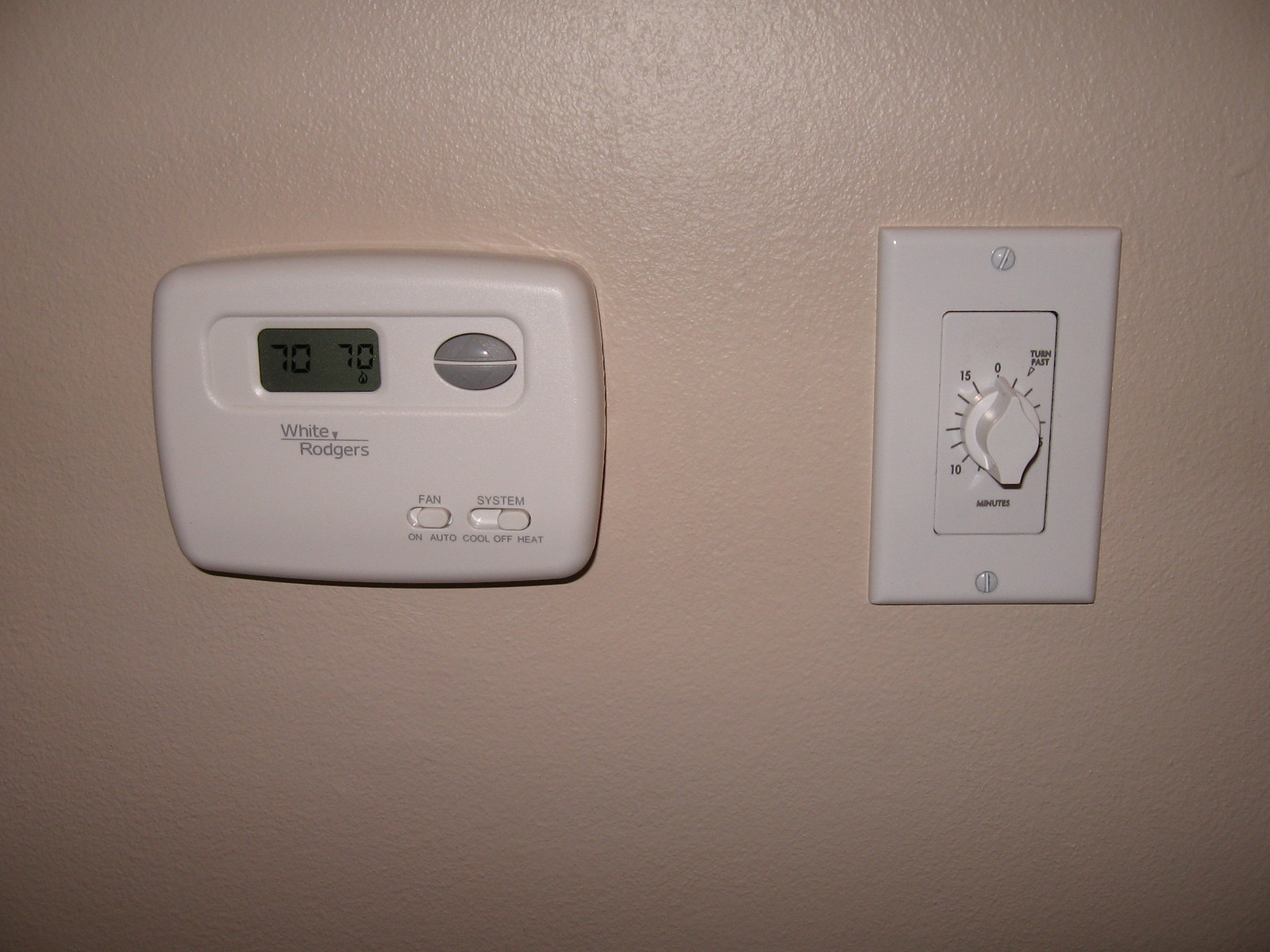In this image, we see two distinct items related to temperature control. On the left, there is a small, white, rectangular thermostat branded by White-Rodgers. The thermostat display shows a temperature of 70 degrees, which likely reflects the desired room temperature setting. The device features two buttons: one with an upward arrow to increase the temperature, and another with a downward arrow to decrease it. Below the display are controls for the fan and system modes. The fan setting can be toggled between "On" and "Auto," with the current setting appearing to be on "Auto." The system control offers options for "Cool," "Off," and "Heat," with the toggle currently set to the "Heat" position.

To the right of the thermostat, there appears to be a separate device resembling a light switch, likely a timer. This timer has a dial marked with various increment settings: 0, 10, 15, and an unclear number. The dial is currently pointed to the zero position, indicating that the timer is not actively set.